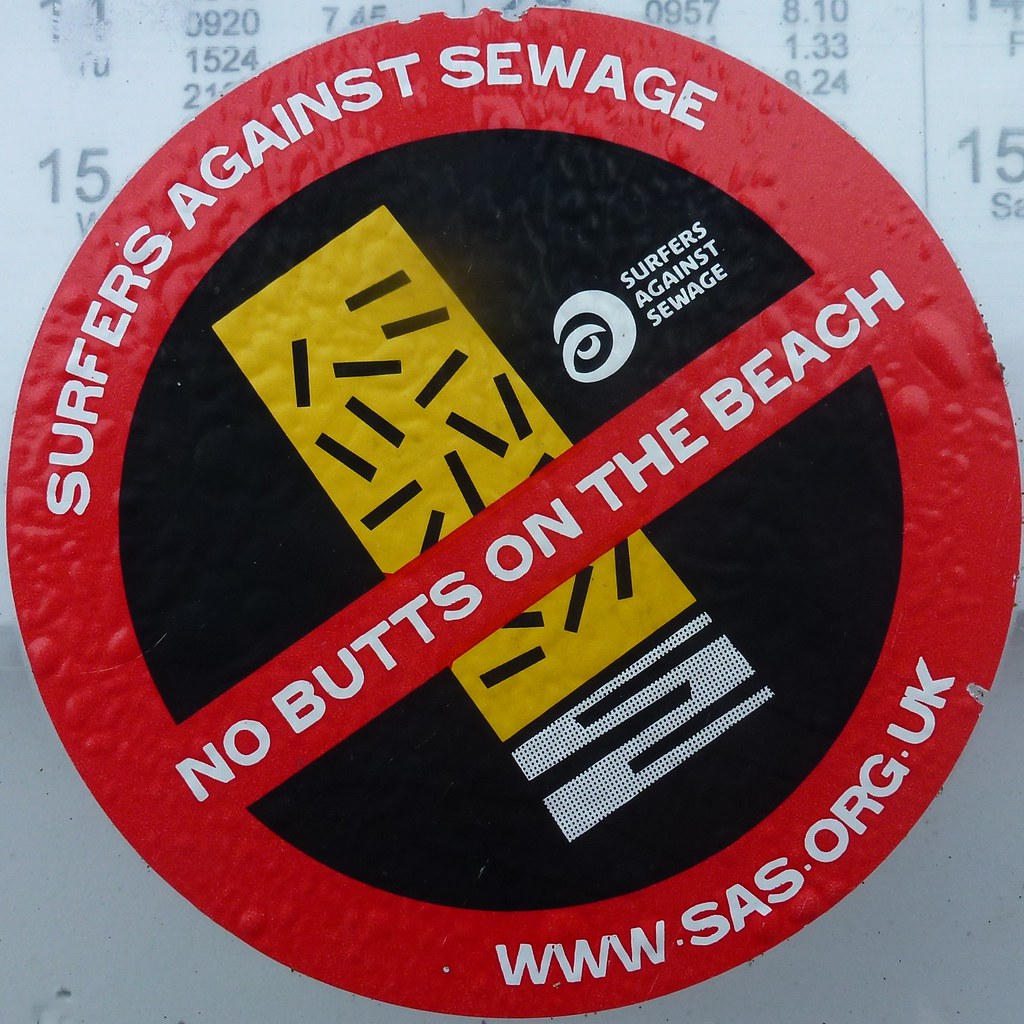In the image, there's a prominently displayed sign that features a large, red crossed-out circle, symbolizing prohibition. Within this circle, there's an abstract depiction of a cigarette with a yellow body and a white tip, resembling the part that is smoked or burned. The cigarette is positioned diagonally across the sign. 

At the top left and bottom of the sign, the phrase "Surfers Against Sewage" is clearly visible, with the organization's website, "www.sas.org.uk," located at the bottom. Inside the circle, there's also a white logo that resembles waves or curves, associated with the Surfers Against Sewage organization. Over the cigarette, the words "No Butts on the Beach" are prominently displayed.

The sign rests on a grayish background, taking up around two-fifths of the bottom part of the image, while the upper part features a white wall. Various numbers, potentially representing dates or a schedule, such as "15," "0 9," "20," "15," "24," and "21," are scattered above the phrase "Surfers Against Sewage."